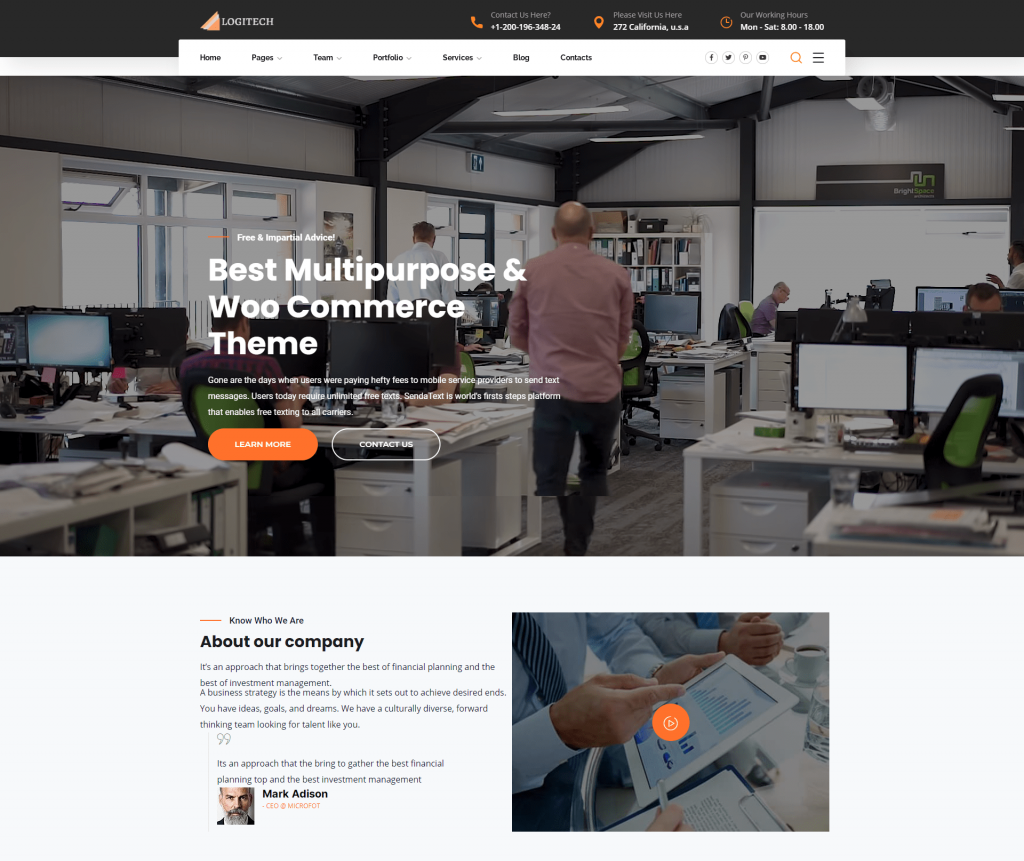The image depicts a detailed webpage from the Logitech website. The company logo is prominently featured, comprising three geometric shapes: two orange triangles and one pink prism. The header section of the page is set against a black background, featuring a clickable phone icon labeled "Contact Us Here" and an address that reads "Please Visit Us Here: 272 California, USA." Also displayed are the working hours: Monday to Saturday, from 8:00 to 18:00.

At the bottom of the page, a variety of navigation tabs are present, including Home, Pages, Team, Portfolio, Services, Blog, and Contact, accompanied by social media icons for Facebook, Twitter, Pinterest, and YouTube. There is also an orange search bar alongside a menu option.

Dominating the center of the page is a prominent white text that reads: "Free and impartial advice. Best multi-purpose and work commerce team." The text elaborates with, "Gone are the days when users were paying hefty fees to mobile devices to send text messages. Users today require unlimited free text. Send a text is the world's first platform that enables free texting to all carriers. Learn more, contact us." 

Below this, a yellow "Learn More" button is available for further information.

Towards the bottom of the page, under "About Company," another detailed text explains the site's approach: "Our approach brings together the best of financial planning and investment management. A business strategy is the means by which our desired ends are achieved. You have ideas, goals, dreams. We have a culturally diverse, forward-thinking team looking for talent like you."